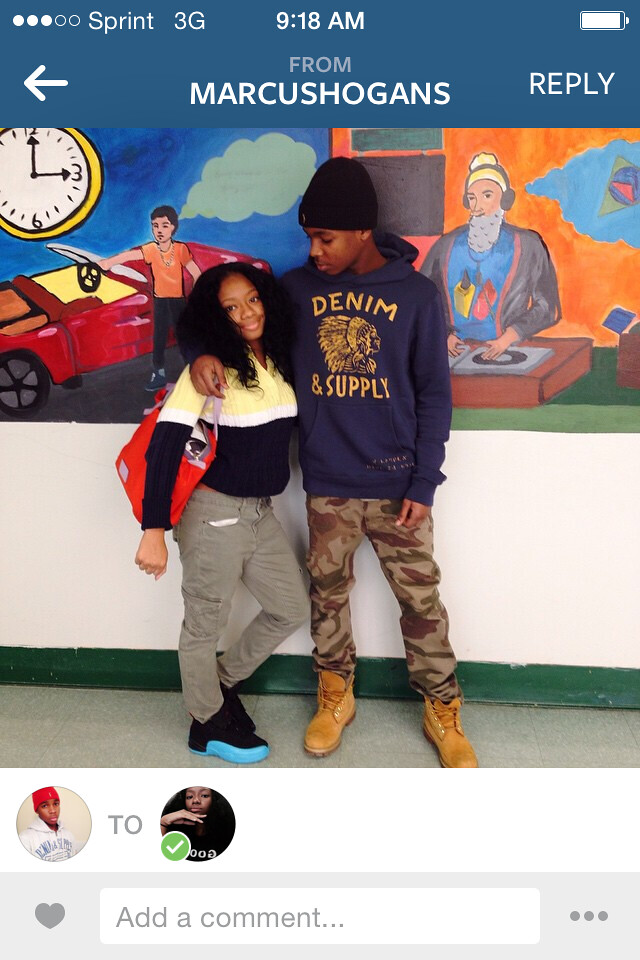This detailed image captures two African-American high school students, a boy and a girl, standing in front of a mural at their school that features significant community artwork. The boy is wearing a black beanie, a blue hoodie with the phrase "Denim Supply" and a graphic of a Native American, brown and green camouflage pants, and a pair of Timberland boots. He has his right arm draped around the girl, who is dressed in khaki pants and the Carmelo Nuggets edition of Jordan 12 shoes. The mural behind them includes vibrant images: a red car with a boy standing next to it, a large clock indicating 3 o'clock, and a DJ with a beard and headphones spinning records on a turntable. This scene was captured in a screenshot from Marcus Shogans’ Sprint phone with a 3G connection, taken at 9:18 a.m., as indicated by the phone's interface details.